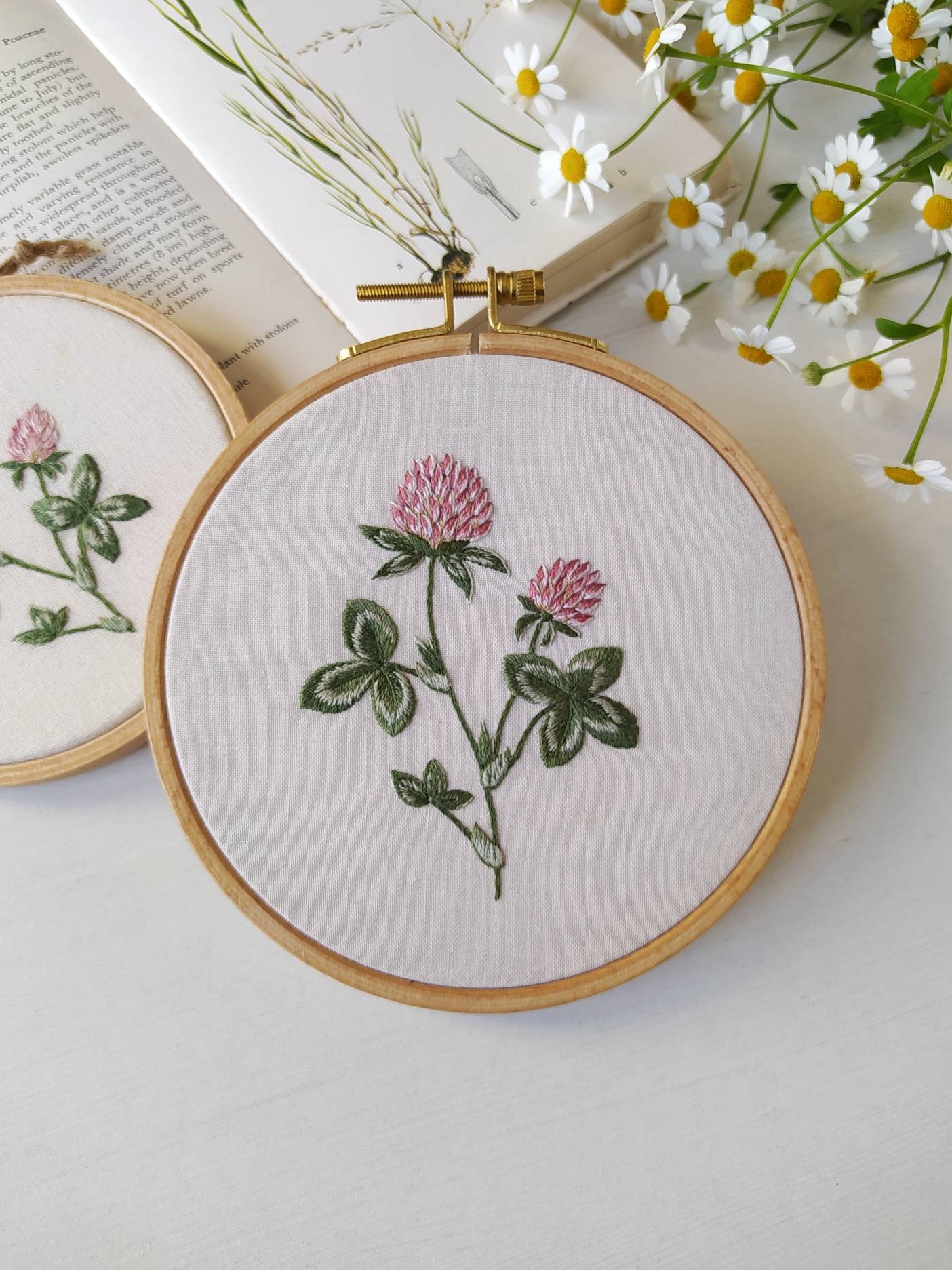This photograph captures a detailed scene featuring intricate needlepoint work placed atop an open book. Central to the image is a prominent needlepoint hoop with a golden screw, keeping the fabric taut. The needlepoint depicts a floral design: a large pink bloom on the left, accompanied by smaller flowers on the right, each arising from a stem flanked by three-leaf clusters. To the side, partially visible, is a second needlepoint piece with a smaller flower that appears less developed. The open book beneath them shows text on the left page and a pencil sketch of leaves and flowers on the right. Nestled at the top right corner of the image is a bouquet of real daisies with white petals and yellow centers, enhancing the overall composition. The backdrop is a pristine white, possibly a tablecloth, that adds to the clean and elegant aesthetic of the scene.